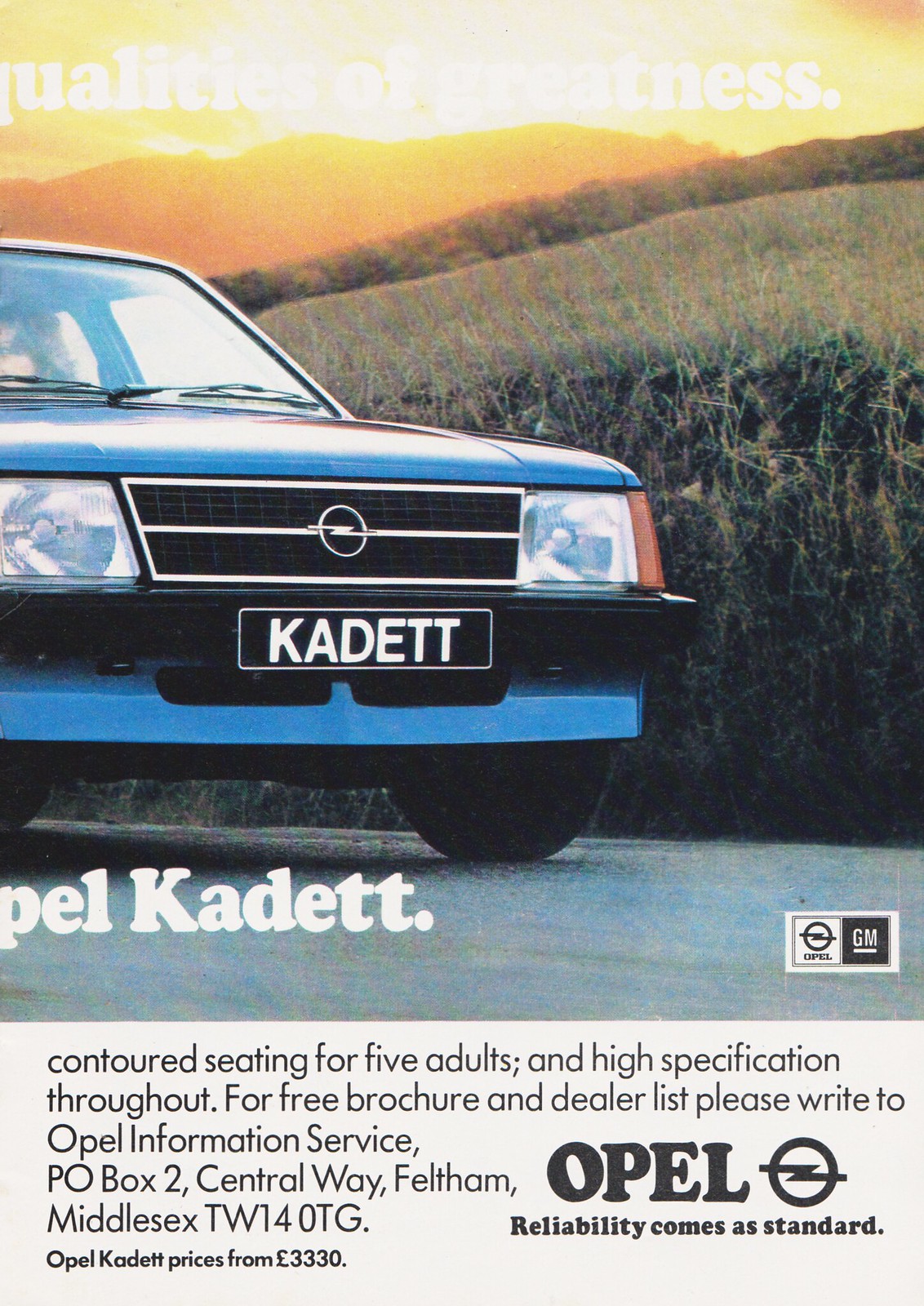This vintage print advertisement, likely from the 1960s or 70s, is for the Opel Kadett, a blue, boxy car prominently featured against a scenic backdrop of rolling hillside and bright sunlight. The image, taking up three-fourths of the vertically rectangular page, showcases the car's front half driving on a road with a logo on the grille—depicting a circle with a lightning bolt—indicating it’s a GM Opel vehicle. The license plate reads "Kadett," and the bottom of the ad includes key details: "Opel reliability comes as standard," "Contoured seating for five adults and high specification throughout," and information on how to get more details: "For free brochure and dealer list, please write to Opel Information Service, P.O. Box 2, Central Way, Feltham, Middlesex, TW14 0TG." The ad also lists the starting price as £3,330.